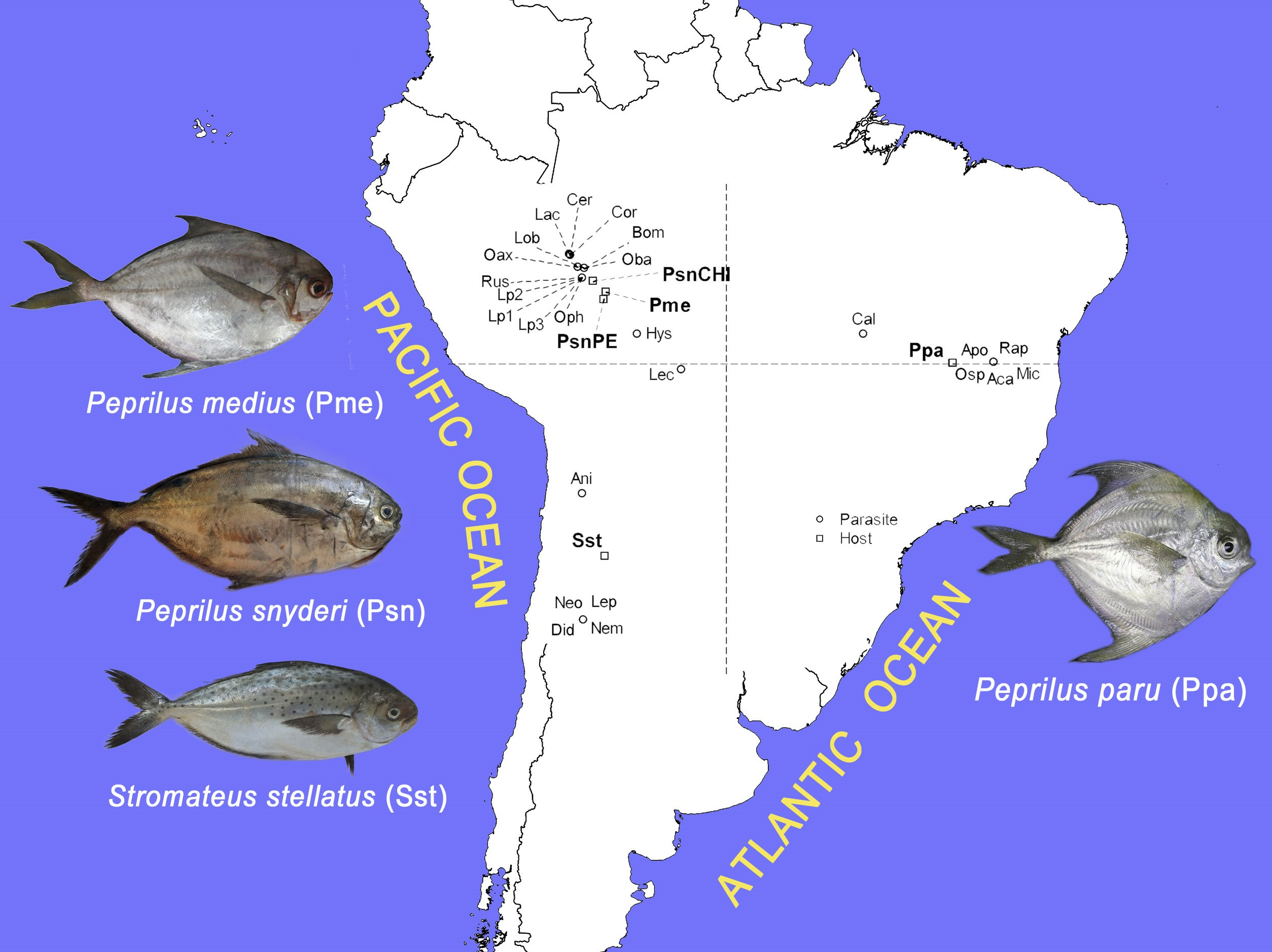The image depicts a computer-generated map of South America set against a lavender background, with photographs of four types of fish superimposed around the continent. The map is minimally detailed, showcasing a white outline of South America, annotated with black lines and specific abbreviations for the fish species. The Pacific Ocean is indicated on the left and the Atlantic Ocean on the right. On the left side of the continent, three silver-gray, finned fish—Paprylis medias (P-M-E), Paprylis cinderi (P-S-N), and Stromatias stellatus (S-S-T)—are vertically aligned from top to bottom, with all fish oriented to the right. To the right, a single fish, Paprylis peru (P-P-A), is shown near the Atlantic Ocean. The fish are tall and narrow, resembling a flounder, and are detailed to illustrate where they are caught, their respective oceanic habitats, and distinctions between parasites and hosts. The predominant colors in the image are the purple background, the silver of the fish, and the white of the continent with black annotations.